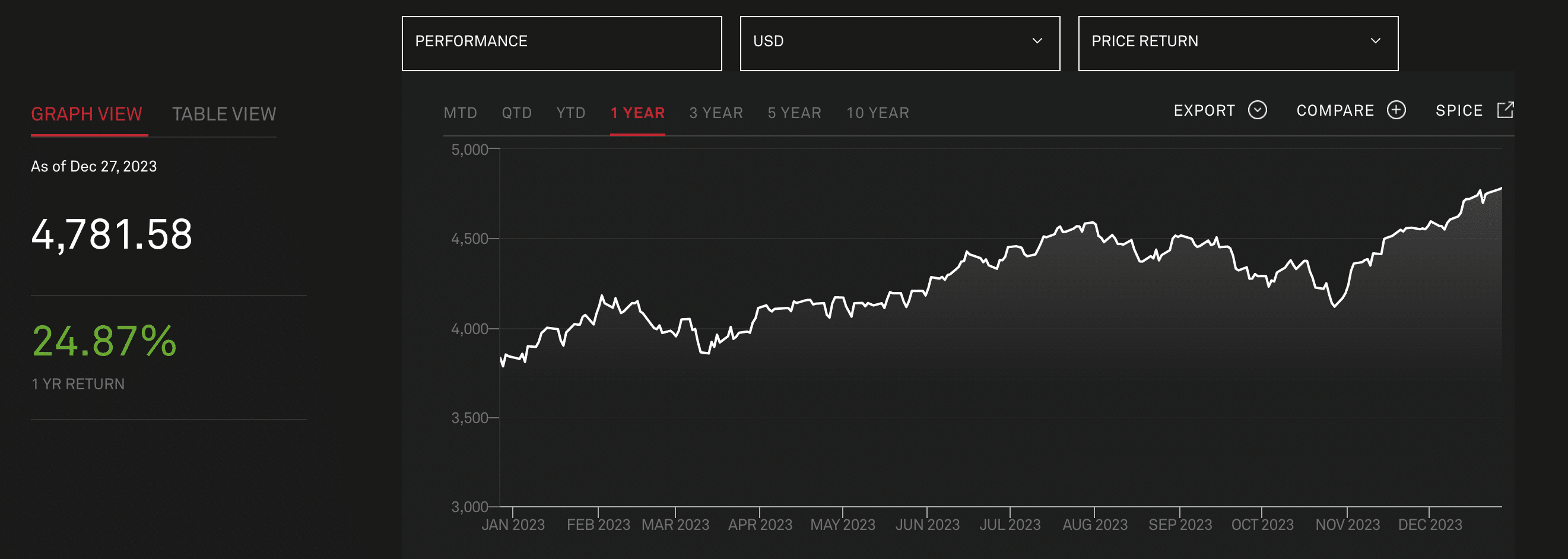The image is a detailed representation of a stock market performance chart with a black background occupying approximately one-third of the left side of the frame. Within this black background, a black square is positioned near the top-left corner. Inside this square, the text "GRAPH VIEW" is displayed in bold red, capital letters about two inches from the top, underlined with a red line. To its right, the words "TABLE VIEW" appear in gray, all capital letters. Beneath these labels, the text "As of December 27, 2023" is written in white.

Dominating the center of the image, the figure "$4,781.58" is prominently displayed in large white text, indicating the current market value. Below this figure, a green percentage, "24.87%", signifies the performance change, specifically labeled as "One Year Return" in smaller white text directly below it.

To the right, three tabs are organized horizontally. The first tab, "Performance in USD," is highlighted in white with a black background and white border. The subsequent tabs feature white text and have drop-down arrows on the right side, indicating additional options.

Below the tabs, performance metrics are listed horizontally in gray text: "MTD" (Month-To-Date), "QTD" (Quarter-To-Date), "YTD" (Year-To-Date), and "One Year," with "One Year" underlined in red indicating it is the selected timeframe. Following these metrics, additional periods, "Three Year," "Five Year," and "Ten Year," are labeled in black text. Further to the right, options to "Export" (marked by a white circle with a check mark), "Compare," a plus icon, a "Splice" option, and a box with an arrow pointing upwards to the right are displayed.

On the left side of the chart, vertical labels indicate values ranging from "5,000" at the top, descending through "4,500," "4,000," "3,500," to "3,000" at the bottom. Along the horizontal axis at the bottom, monthly labels from "January 23" on the left to "December 23" on the right span the width of the chart. A fluctuating line graph, starting just below the "4,000" mark, illustrates peaks and valleys of stock market performance, gradually rising and falling across the year, reaching approximately the "4,750" mark in December, visually depicting the market's upward and downward trends over the year.